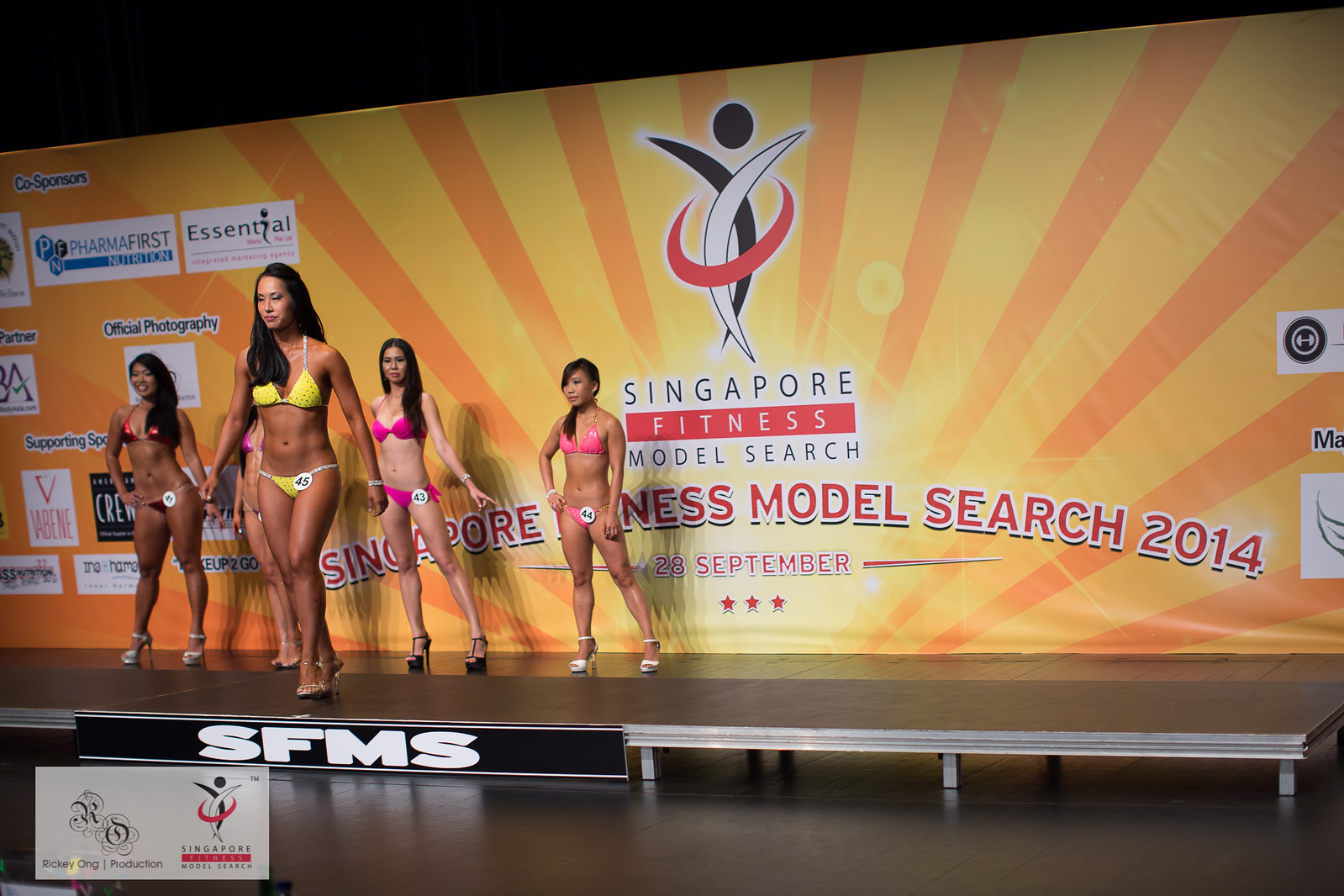This image depicts a scene from the "Singapore Fitness Model Search 2014," held on September 28th. Five female contestants, all wearing bikinis with numbers clipped to the bottom pieces, stand on a slightly elevated black stage. The numbers visible include 41, 43, 44, and 45, with contestant number 45 in a yellow bikini positioned at the front center. The backdrop features vibrant orange and yellow sunburst stripes with the event’s title prominently displayed. To the left side, a collection of sponsor logos—though some are partially obscured or fuzzy—are visible, including Pharma First Nutrition, Essential, Official Photography, and Ricky Ong Productions. The acronym "SFMS" is marked at the front center of the stage.